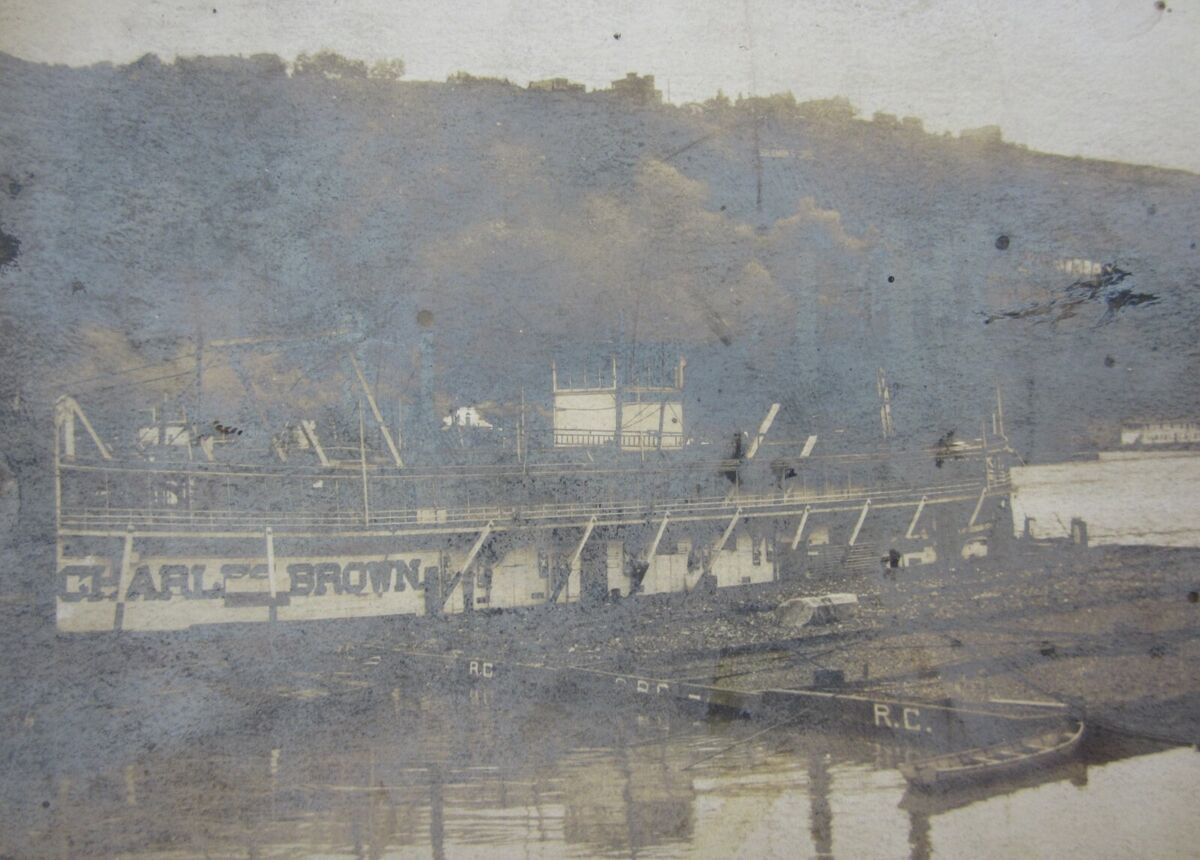This aged sepia-toned photograph, shrouded in a hazy film possibly due to its age, depicts a vintage World War II-era ship—likely a battleship—bearing the name "Charles Brown" or possibly "Charlie Brown" in large dark letters on its white bow. The ship is anchored in a murky, dirty river, stretching horizontally to occupy nearly the entire image frame. Accompanying the ship are smaller vessels labeled "RC," which appear to be rescue crafts, such as lifeboats. The scene is set against a tranquil backdrop of trees adorning a small hill or mountainside. Dotting the image, faint scratches and blemishes reveal the photo’s considerable age, adding to its historical ambiance.